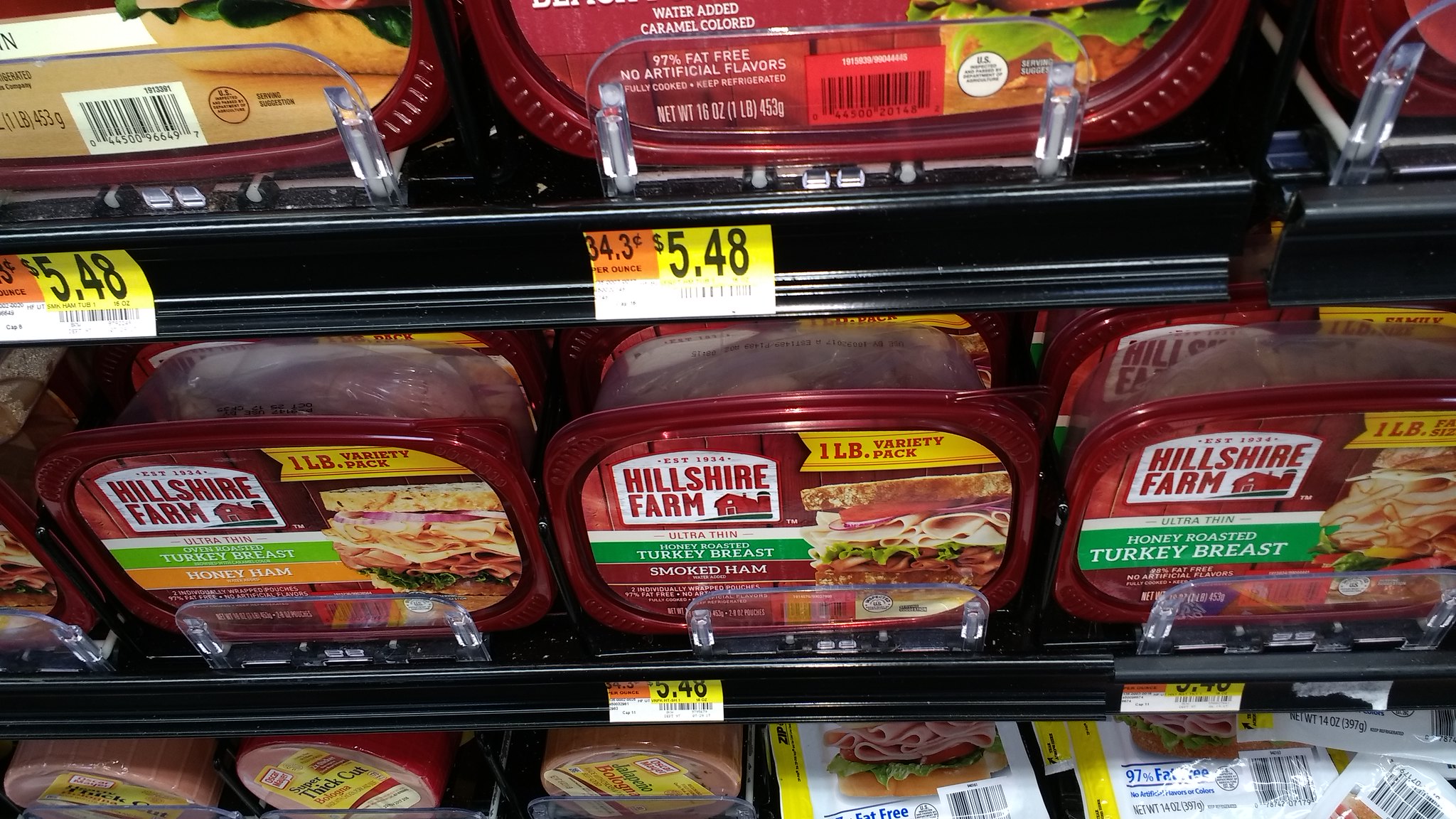This image, taken at Walmart, depicts a close-up of the refrigerated deli section showcasing various packaged deli meats. The distinct Walmart price tags are visible, with a bright yellow section indicating the price of $5.48 and an orange box on the left showing the cost per ounce, listed as 34.3 cents. The products are primarily Hillshire Farm varieties, identified by their clear plastic tubs with red tops. The shelves display a variety of deli meats, including a one-pound Hillshire Farm variety pack containing turkey, salami, and honey ham, along with packages of turkey breast and smoked ham. There are also packages of honey roasted turkey breast in different forms, such as a small can. Beneath the main products are other deli meats, which include bologna and possible Carl Buttig small packets. The overall organization showcases a well-stocked deli section, marked by consistent packaging and clear pricing for easier comparison.